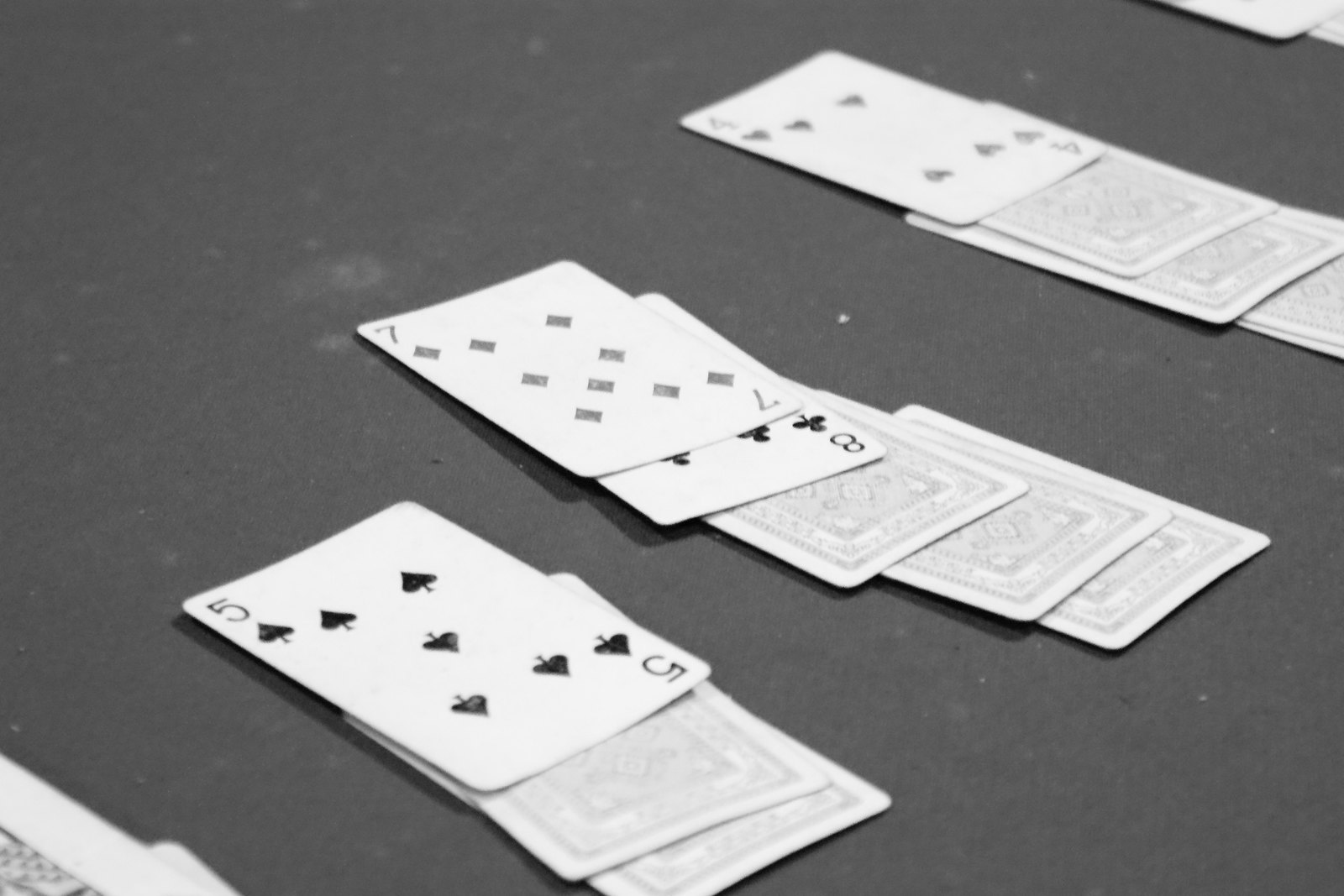A black and white photograph captures a moment in a solitaire game on a black felt board. The surface shows signs of use, with visible stains near the seven of diamonds and small white specks scattered across the backdrop. In the composition, a four of hearts, seven of diamonds, and five of spades are prominently displayed, indicating the early stages of the game. Additional columns of cards are faintly visible in the upper right-hand corner, suggesting the initial layout of the tableau. To the lower left, another object or image with white elements intrudes slightly into the frame. The absence of hands or a visible player gives the scene a somewhat solitary and timeless quality, reinforcing the solitary nature of the game.